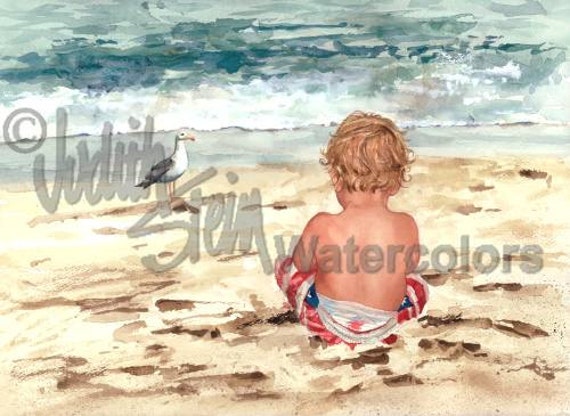This detailed watercolor painting by Judith Stein, prominently watermarked with "Judith Stein Watercolors" and a copyright symbol, captures a serene beach scene from behind a young boy, approximately three to five years old, sitting cross-legged on the sand. The child, with curly blonde hair that reaches his ears, is depicted wearing patriotic red, white, and blue swim trunks reminiscent of the American flag, with a hint of a diaper peeking out from the back. He is gazing out over the ocean, which features gentle waves breaking along the shore, with a palette of blues, greens, and frothy whites. Beside him to the left, a white seagull with gray wings and a yellow beak stands, seemingly gazing at the child. The sandy beach is portrayed in varying shades of tan, yellow, and brown, suggesting footprints that hint at past activity. Above the water, the sky is filled with gray clouds, adding to the tranquil and contemplative mood of the scene. The illustration is devoid of other people or structures, enhancing the focus on the boy and his lone companion, the seagull, against the expansive maritime backdrop.